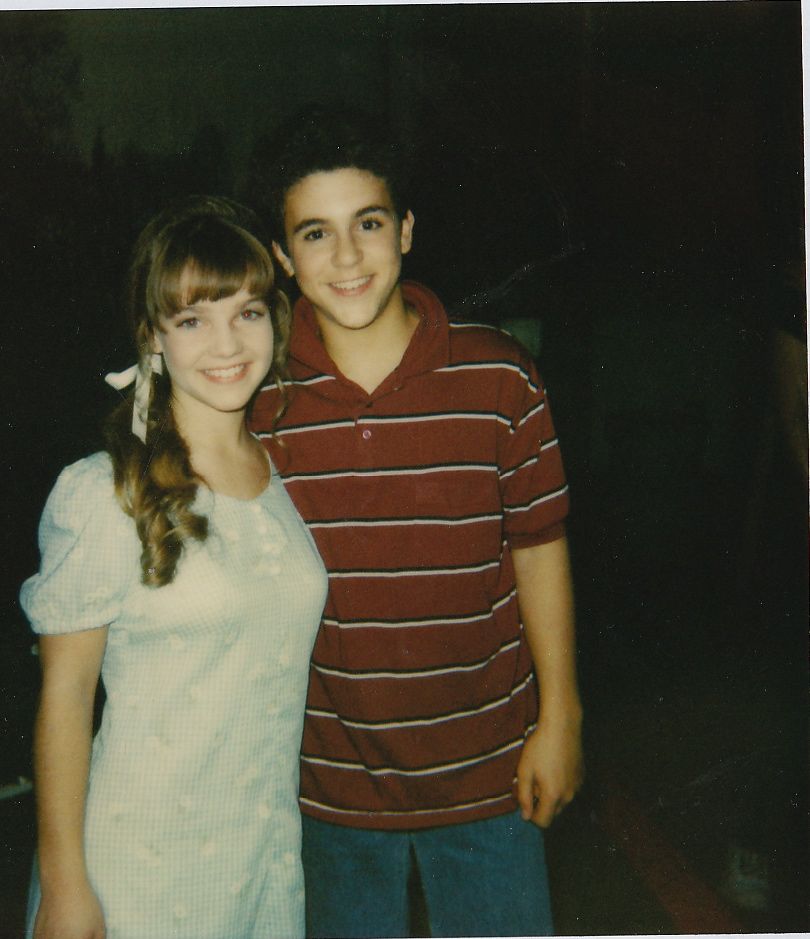The image depicts two young teenagers, possibly around 13 or 14 years old, standing in a dimly lit room and posing for a picture. On the right, a boy with dark brown hair, who might be Ben Savage or his brother, is smiling. He’s dressed in a red polo shirt adorned with thin black and white stripes and paired with blue jeans. On the left stands the girl, who has medium brown hair styled in curls at the bottom, accented with white bows. She’s wearing a white dress and also smiling. She appears to have red-eye effect from the camera flash. The boy is slightly positioned behind the girl, and the overall ambiance of the room is dark, making other background details hard to discern.